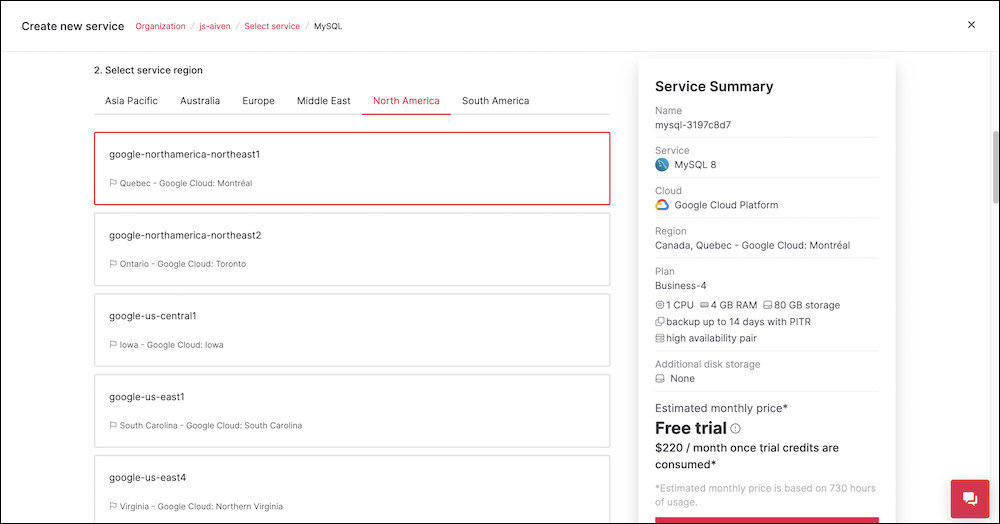A detailed screen capture showcases a web interface for creating a new service. The background is predominantly white, with mixed red and black text at the top. The heading reads "Create New Service" and below it, the organization is listed as "JSAVEN." Following this, it instructs to "Select Service," showing "MySQL" as the choice. 

A thin gray line separates this section from the rest of the content. Above the line on the right is a gray 'X' icon, likely for closing the panel. Below this line, the text "Select Service Region" is displayed in gray. The regions listed include "Asia-Pacific," "Australia," "Europe," "Middle East," "North America," and "South America." "North America" is highlighted in red and underlined.

Further down, several white boxes with black text are visible. The first box, highlighted in red, reads "Google-North America-North East 1," accompanied by a small flag icon. Below this, the entries are:

- "Google-North America-Northeast 2," flagged and listing "Ontario, Google Cloud Toronto."
- "Google-US-Central 1," flagged and listing "Iowa, Google Cloud Iowa."
- "Google-US-East 1," flagged and listing "South Carolina, Google Cloud South Carolina."
- "Google-US-East 4," flagged and listing "Virginia, Google Cloud Northern Virginia."

Another white box further down displays a "Service Summary." It reads:
- "Name: MISCI" followed by a unique string of letters and numbers.
- "Service: MySQL 8" with a teal icon next to it.
- The Google Cloud Platform logo, which is red, gold, and blue.
- "Region: Canada, Quebec, Google Cloud Montreal."
- Additional details include "planned business 4," "one CPU," "4 gigabytes of RAM," "80 gigabytes of storage," "backup up to 14 days with PITR," "high availability payer," "additional disk storage: none," "estimated monthly price: free trial or $220 a month once trial credits are consumed," and "estimated monthly price based on 730 hours of usage."

At the bottom, there's a pinkish-red bar, and within this section, a red box with a white bubble is present.